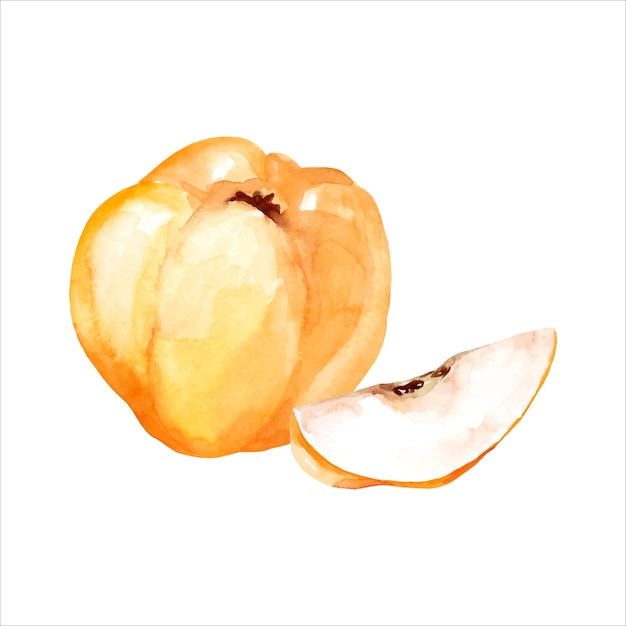This image is a detailed color illustration in a square format depicting a yellow apple with orange highlights against a white background. Central to the illustration is an unevenly circular apple, displayed prominently on the left side. A slice has been removed from the apple and is placed to the right, with its cut edge facing upwards. The slice reveals the white flesh and several small, dark seeds in the center. The main apple features a central stem area that is slightly recessed and topped with a dark, spiky structure. Despite its vibrant yellow and orange hues, the fruit's irregular, lumpy texture and the shading give it an almost unappealing appearance, reminiscent of a slightly deteriorated or bruised apple. The illustration is bordered by a light gray rule.